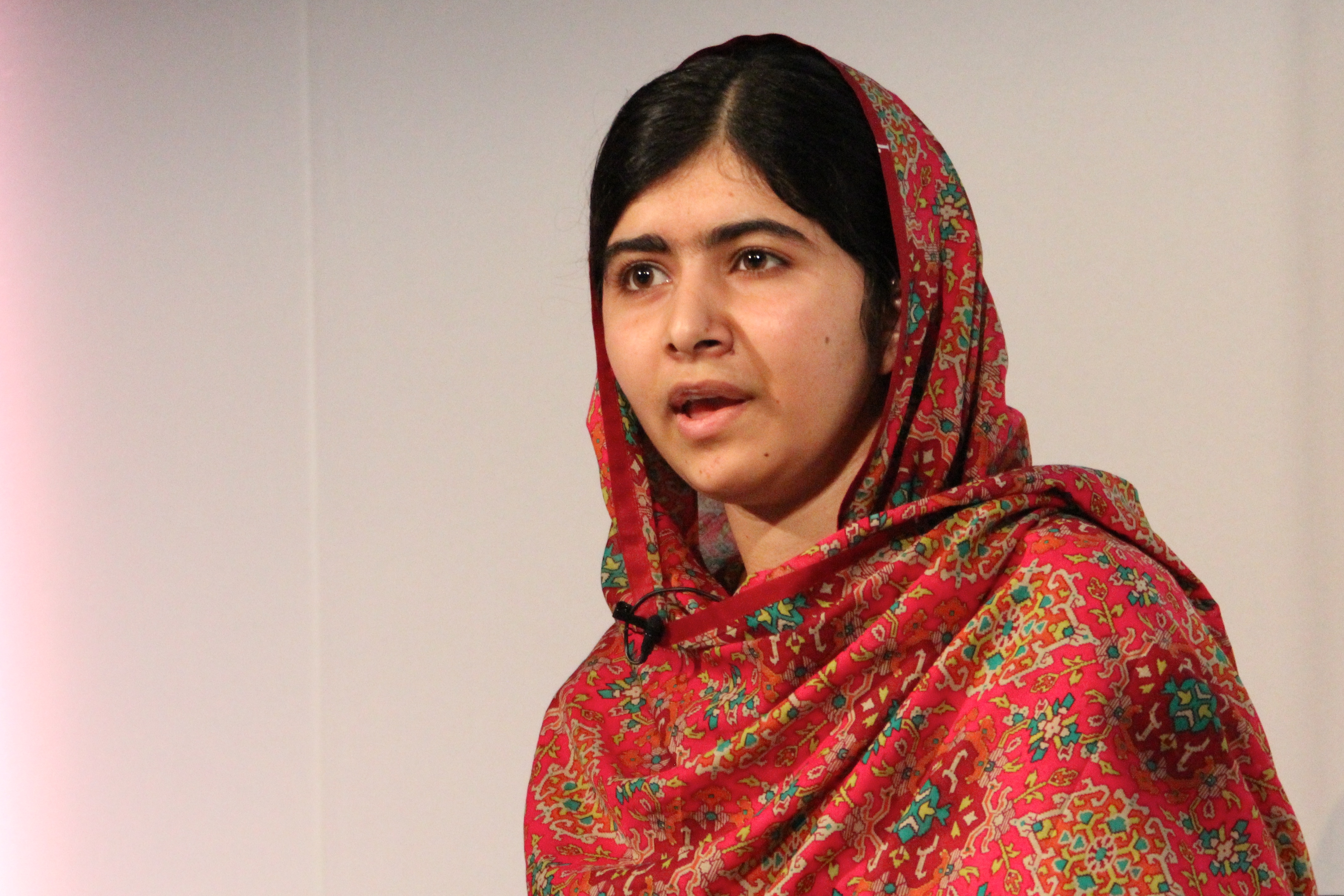Against a vibrant pink background, an image captures a woman of apparent Indian descent, centered within the frame. She is adorned in a coordinated red outfit featuring a head covering that seamlessly flows into a shawl draping over her shoulders and chest. The fabric is intricately patterned with green and orange designs accented by white and yellow details, including alternating green circles and yellow triangles. Her long black hair, parted in the middle without bangs, peeks out from under the head covering and cascades down her back. The woman, with her brown eyes and slightly parted lips indicating she might be speaking, gazes towards the left side of the image (her right). A notable detail is the subtle presence of a microphone clip attached to her garment, hinting at her potential involvement in a speech or presentation.